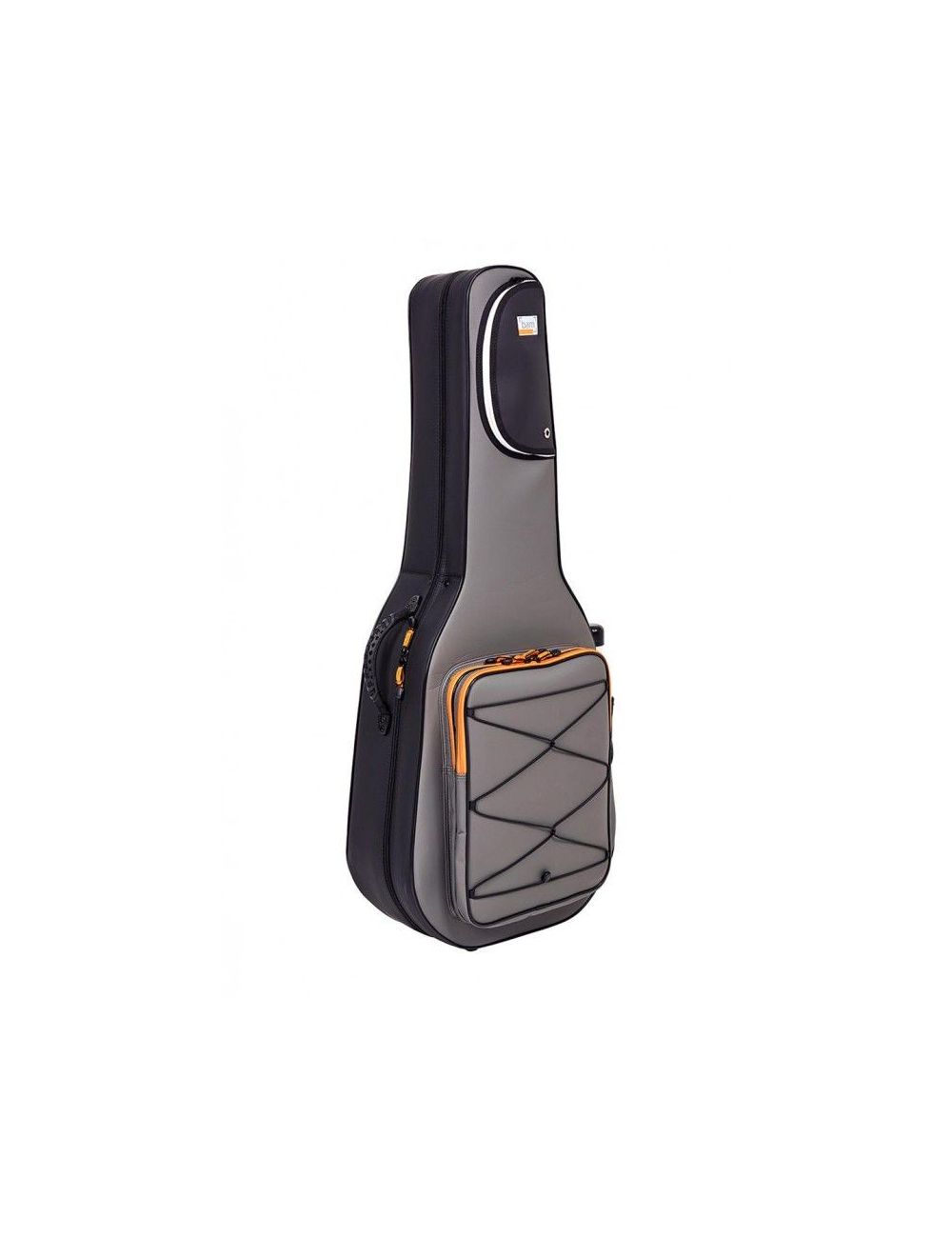The image depicts a modern guitar case standing upright against a plain white background with no visible borders. The case is predominantly gray, with the front portion being a lighter shade and the sides a darker gray. The left side of the case faces slightly towards the viewer, revealing a dark gray section where a black handle is located halfway down. The zipper lines, which feature orange-yellow detailing, run along the sides. The front of the case includes a rectangular bottom pocket characterized by a distinctive zigzag black design forming geometric shapes such as triangles and diamonds. This pocket also has green zippers and a crisscross pattern of elastic bands on its surface. The top of the case features a small half-circle pocket in dark gray, outlined with a black, white, and black border, and includes an unreadable rectangular tag. The overall construction of the case suggests it is sturdy and well-made, suitable for a guitar, with plastic and fabric materials providing durability.